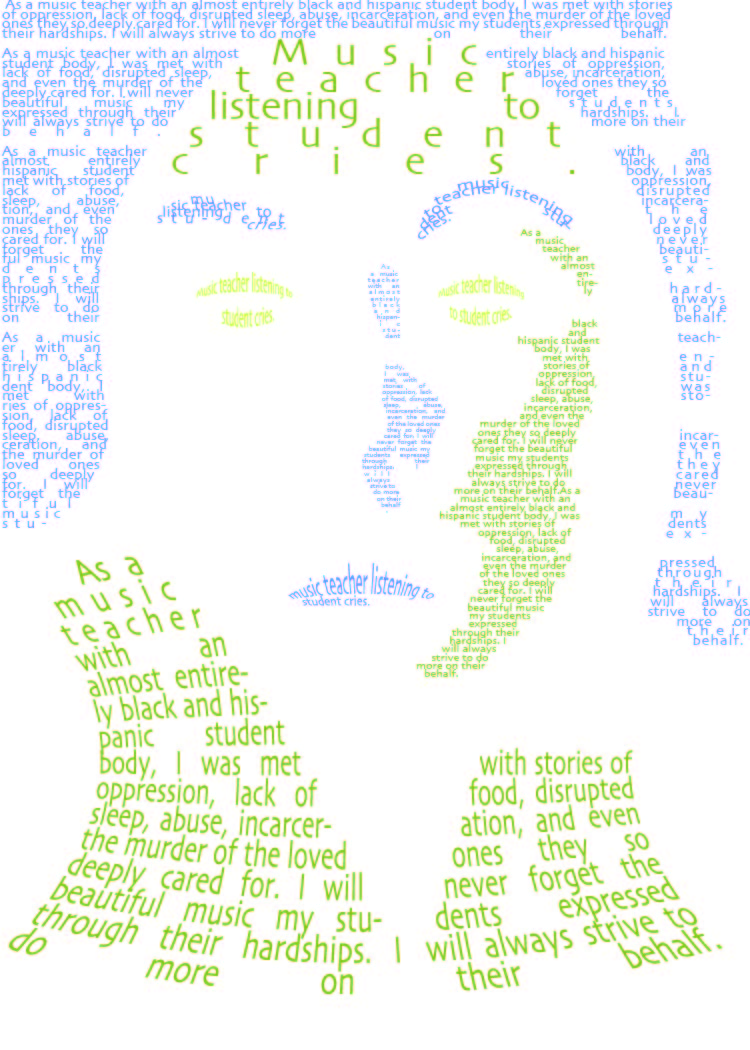The image is a detailed portrait of a face constructed entirely from various-sized words and colored text. In the center of the image, the face is formed with an intricate arrangement of text, creating distinct facial features such as eyebrows, eyes, a nose, and a mouth. The colors used for the text include lavender, light green, dark green, and white, adding depth and dimension to the portrait.

At the top of the head, larger text in green reads, "music teacher listening to student cries," while smaller text shapes the forehead and eyebrows. The eyes are crafted from text lines arched above and below, and the nose and mouth follow similarly intricate text formations.

Moving toward the neck, the text forms detailed paragraphs, with one notable section reading, "as a music teacher with almost entirely black and Hispanic student body, I was met oppression, lack of sleep, abuse, incarnate, incarceration, the murder of the loved, deep care." This text in the lower part of the image curves slightly, giving the appearance of a neck and shoulders.

Overall, the face is surrounded by blank space and interspersed with passages of varying text colors and sizes, contributing to the artistic representation of a face made solely from words. The text also forms additional elements like hair and shirt collars, enhancing the portrait’s realism through word-crafted shadows and details.